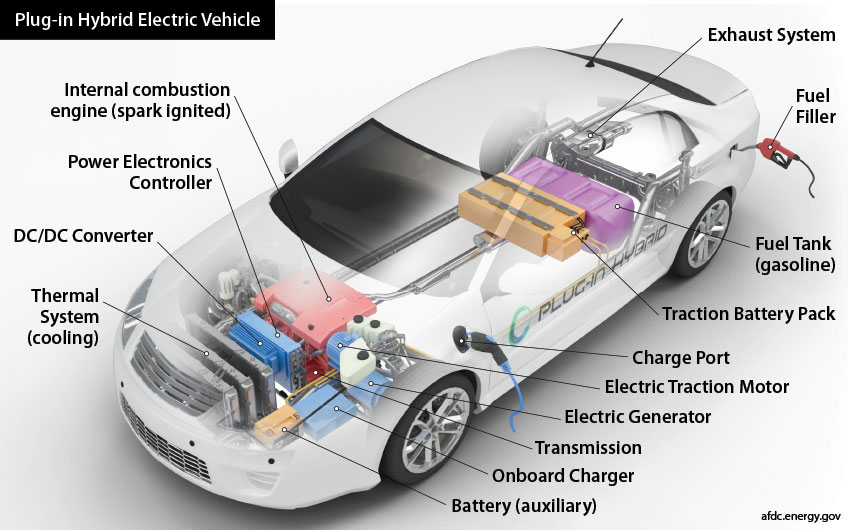The image displays a transparent white car, providing a detailed view of its internal components and mechanisms. Emphasizing its hybrid nature, the top left corner features a black rectangle with white text that reads "Plug-in Hybrid Electric Vehicle." The transparency allows for an intricate look at both the electronic and combustion elements within the car. 

Highlighted with lines and bullet points around the graphic are the key components starting from the top left and moving clockwise: the internal combustion engine (spark-ignited), exhaust system, fuel filler, fuel tank (gasoline), traction battery pack, charge port, electric traction motor, electric generator, transmission, onboard charger, auxiliary battery, thermal system (cooling), DC/DC converter, and power electronics controller. 

This comprehensive layout showcases how the plug-in hybrid system integrates electric vehicle charging capabilities with a conventional combustion engine, providing a clear understanding of the dual power sources and their respective components within the vehicle's structure.